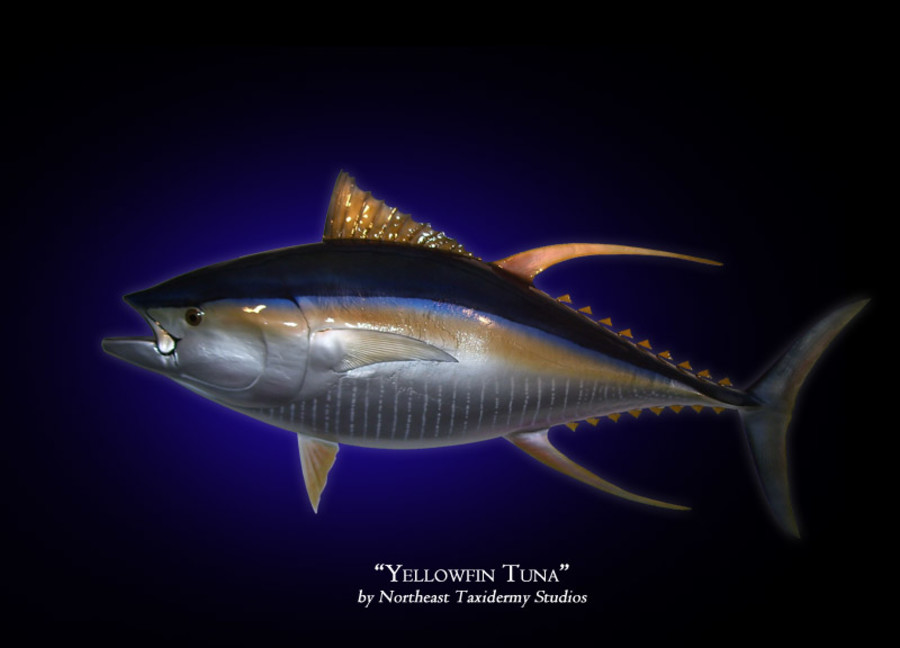The image features a large, colorful yellowfin tuna facing left against an oval-shaped blue background with a dark purple perimeter. The tuna's body displays vibrant hues of blue on its back, transitioning to a silver underbelly, with a distinctive yellow stripe running along its side and a prominent yellow dorsal fin. The fish's mouth is open, and it boasts multiple sharp fins: a top fin, two side flippers, and additional fins near the bottom, with sharp scales towards its tail. Underneath the fish, white capitalized text reads "Yellowfin Tuna" in quotes, followed by "by Northeast Taxidermy Studios." The display suggests the fish has been expertly preserved by the taxidermy studio.